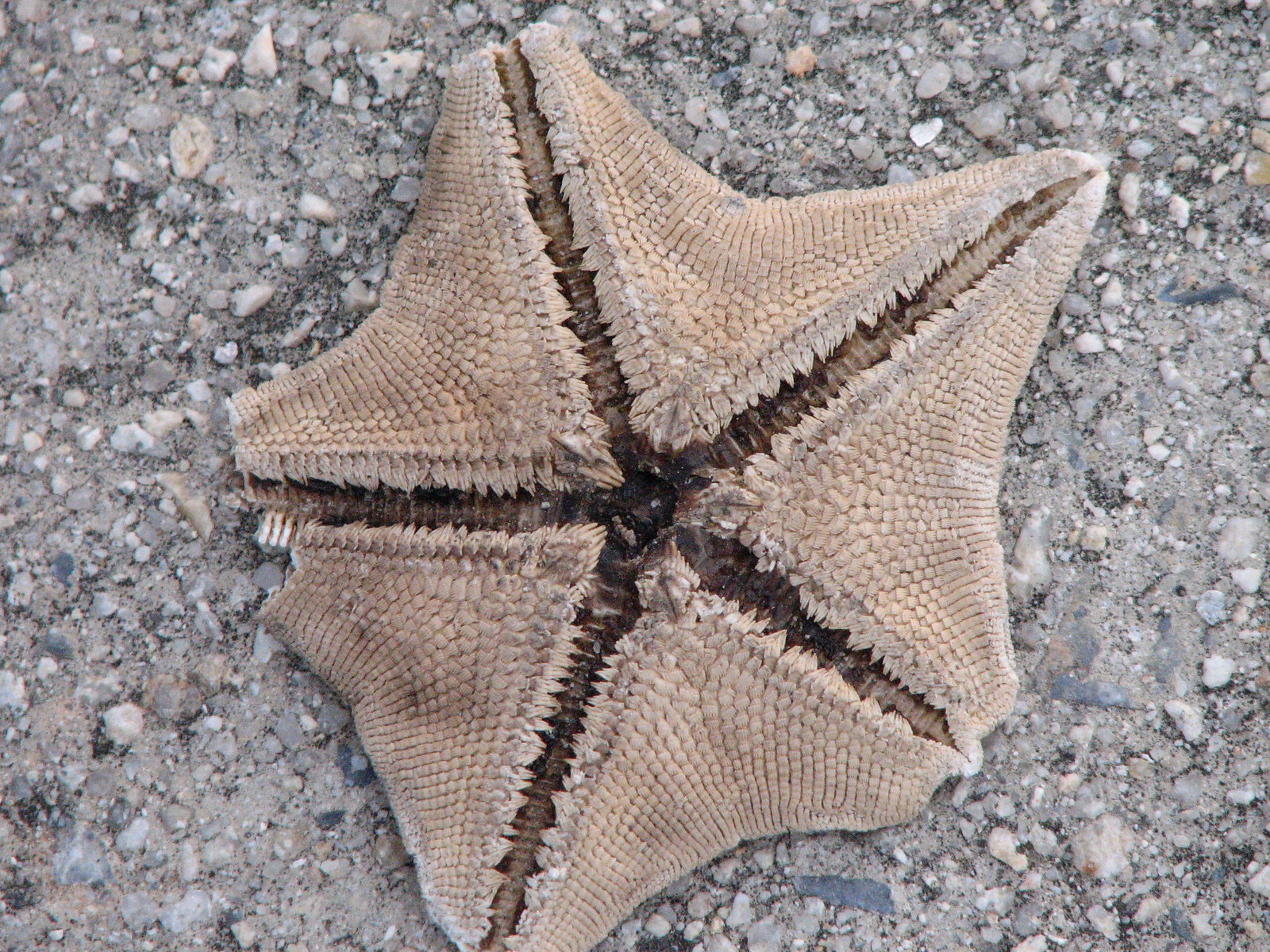The image depicts a starfish situated on a beach characterized by wet, clumpy, and pebble-strewn sand. The starfish, which appears to have weathered significant hardship, occupies the center of the image, displaying a light brown or beige color. Notably, only one of its five points is fully intact—the upper right one—while the other points are chipped away with broken ends, giving the starfish an incomplete appearance. The underbelly of the starfish, featuring a darker brown center, is prominently visible, suggesting possible damage or wear. The close-up nature of the photo emphasizes the imperfections and the possibility that the starfish may no longer be alive, providing a poignant focus on its condition amidst the rugged beach landscape.